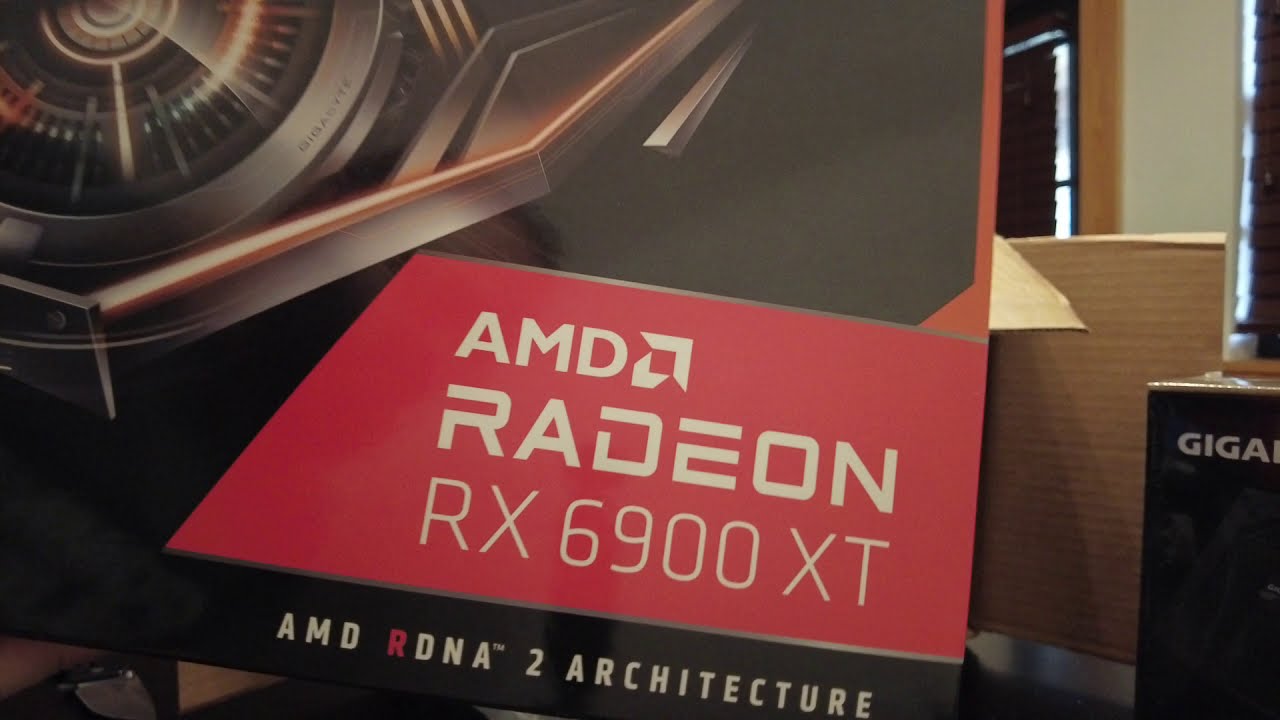The image is an indoor close-up photo of the lower right corner of a product box featuring detailed branding elements. Prominently displayed on the box in white font over a red background are the words "AMD Radeon RX 6900 XT," with "AMD RDNA 2 architecture" written in smaller white text over a black background below it. The box appears to be silver in color, with a metallic swirl or sharp-edged design, somewhat resembling a mechanical part.

Next to this main box is another, likely cardboard, and partly visible is another box with "Giga" on its side. In the background, two windows with closed blinds and a light-colored wall are partially visible, suggesting the setting might be someone's home or an office, though the exact location remains ambiguous due to the tight framing of the photograph. The surrounding environment also includes light wood elements.